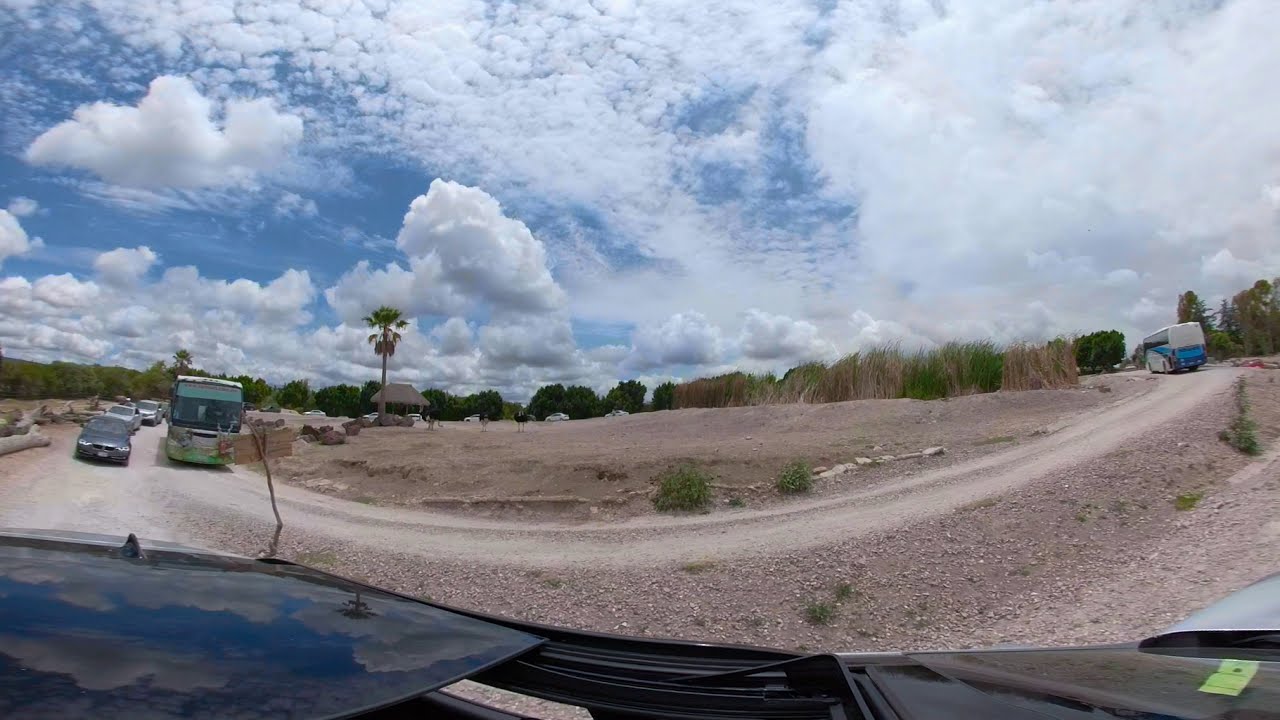The image showcases a panoramic view of a desolate desert area dominated by a dirt-gravel road that swings in a circular motion across the scene. The sky above is filled with a scattering of clouds. Centrally, the barren landscape is marked by a mix of dirt and gravel, encircled by patches of tall grass, predominantly brown with some green on the right side. On the left, an array of vehicles—including a green bus and several cars—are parked or possibly moving slowly along the roadside. There's a hint of a tiny, blurry animal, potentially a camel, in this section of the image. Palm trees and other green trees are visible in the background, with small bushes and occasional weeds dotting the foreground. The image is taken through the sun screen of a black car, adding a shaded frame to the scene, and further to the right, another bus with white and blue stripes can be seen driving along. The overall setting resembles a parking lot or a roadside pullover spot amidst the arid terrain.